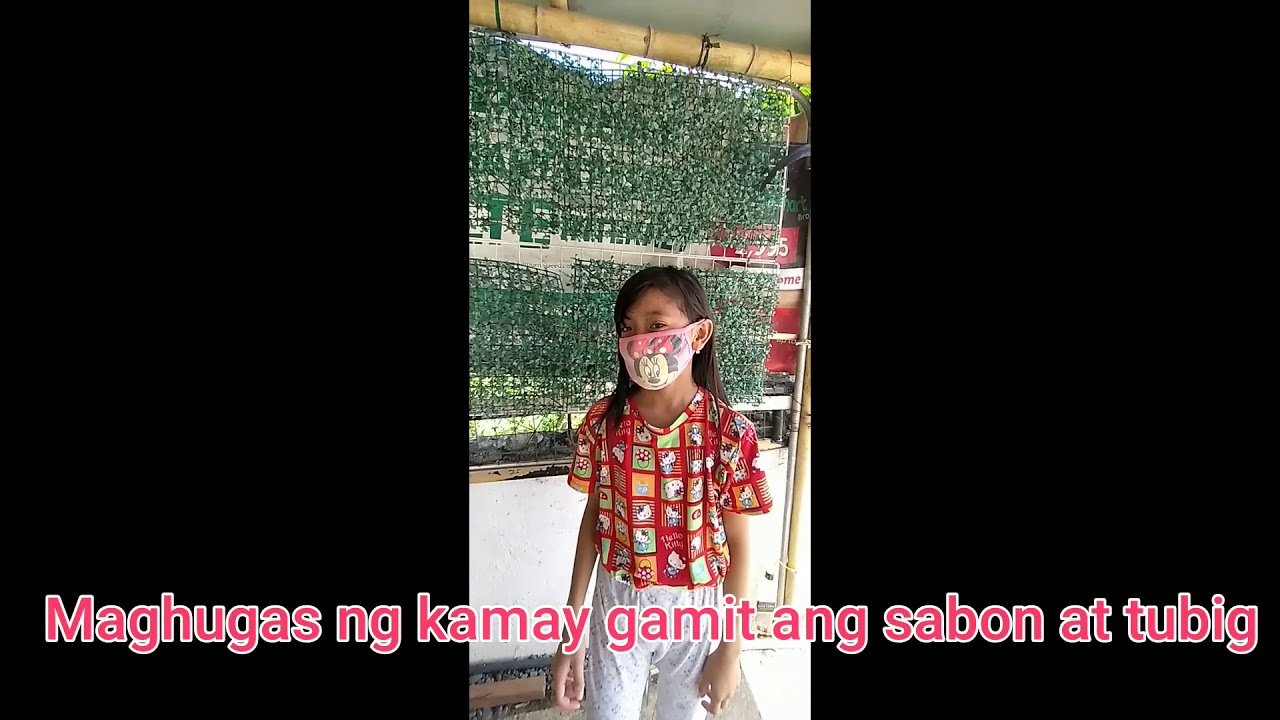The image features a young girl standing beneath an open-air ceiling. She has long black hair and wears a mask adorned with a Mickey Mouse design. Her outfit includes a red shirt with various square patterns and white pants. Behind her, there's a bamboo frame supporting a partially see-through sheet made from a green material resembling fake leaves or camouflage. The area around her appears open but is overshadowed by the black borders, creating a thin central strip for the image. The backdrop also reveals a red metal structure with writing, while across the image, there is text in Indonesian or a similar language, stating "Mahoogas Ng Kamei Gamit Ang Sabon at Tubig" in pink letters with a white outline. The ground behind her is brightly illuminated, adding contrast to the scene.